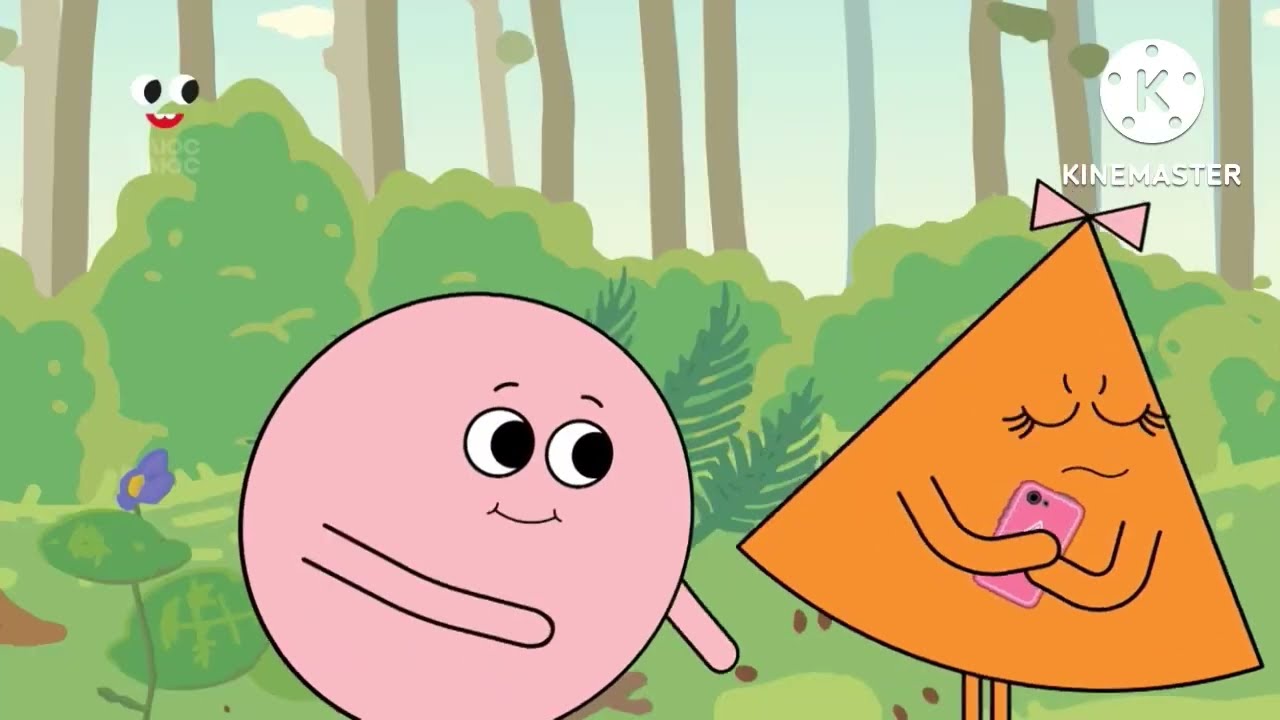In this vibrant cartoon scene likely intended for children, two colorful characters take center stage against a lush, animated backdrop featuring green bushes and distant trees under a partly cloudy sky. Positioned almost directly in the middle of the image, the characters include a grumpy orange triangle on the right, distinguishable by its curvy base, straight legs, and a pink bow atop its point. Hugging a pink iPhone tightly, the triangle displays a frustrated expression with squiggly mouth, closed eyes, and distinct eyelashes. To the left, a cheerful pink circle character with large black-dotted eyes and a beaming smile appears to be engaging with the triangle. The whimsical setting is complemented by an additional detail: a purple flower on the left side. The only textual element visible is the "Kind Master" logo in the top right corner, written in white inside a circled "K". The overall scene, rendered in a playful and colorful style, suggests an educational context, potentially aimed at young viewers learning about shapes.